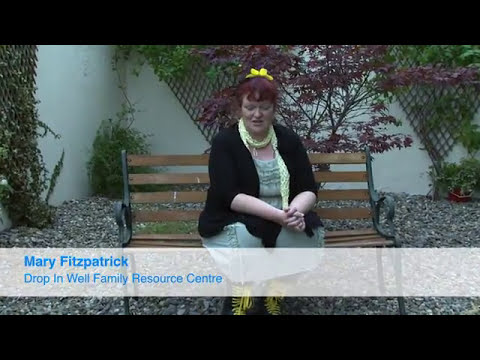In the photograph, which seems likely to be a TV ad for the Drop-In Well Family Resource Center, a woman named Mary Fitzpatrick is prominently featured. A translucent white banner spans the bottom 10-25% of the image, displaying her name and the name of the resource center in light blue text. Mary, a red-haired, Caucasian woman, is centrally seated on a brown wooden park bench. She’s wearing a black, three-quarter sleeve top and a light green dress, paired with black boots that have yellow laces. A yellow ribbon adorns her hair, and she has a small, light green scarf around her neck. She sits with her hands clasped together on her lap, facing the camera. The setting appears to be an outdoor area with wood chips and landscaping stones. The backdrop includes an off-white wall equipped with a wooden lattice supporting climbing plants, an ivy-covered tree on the left, and a small tree with dark purple leaves situated near her left shoulder.